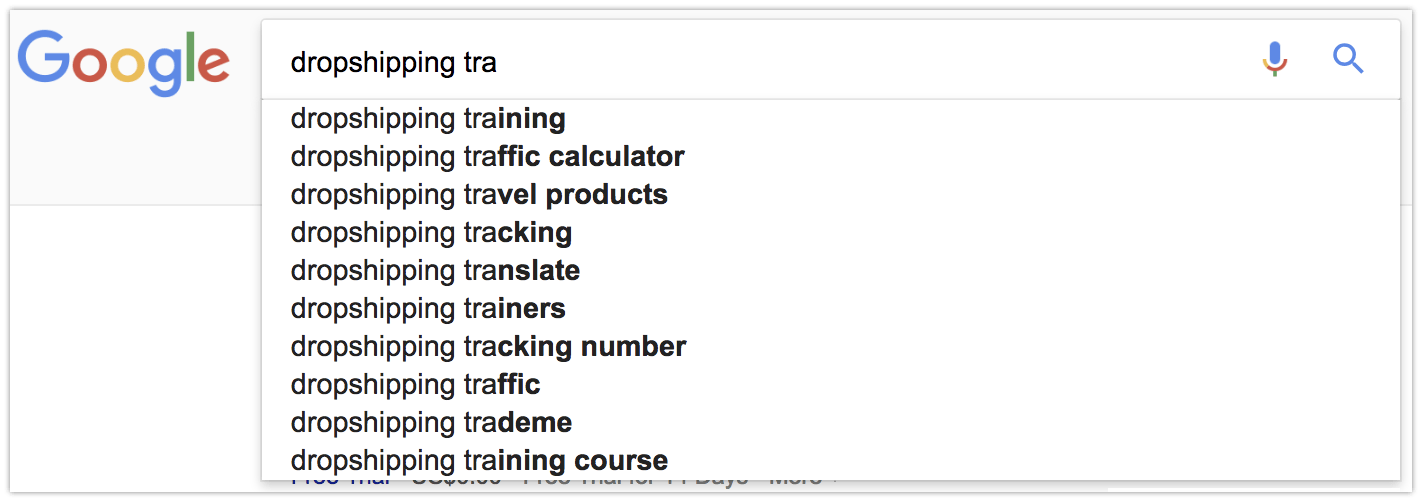The image depicts a Google search page featuring a thin light gray border framing the interface. In the top left corner, there is a light gray box displaying the iconic Google logo in its signature colors: green, red, yellow, and blue. This is set against a very light gray background.

Below the Google logo, a white rectangular search box is positioned prominently. To the right of the search box is a microphone icon and a magnifying glass icon, signifying voice search and standard search functions, respectively. Above the thin gray line that horizontally spans the width of the search box, the text “Dropshipping TRA” is typed in.

Beneath the search box, a list of Google’s search suggestions related to the partially typed query is visible. The suggestions include phrases such as "Dropshipping Trainer" and "Dropshipping Traffic Calculator." The overall layout is clean and minimalist, adhering to Google’s typical user interface design.